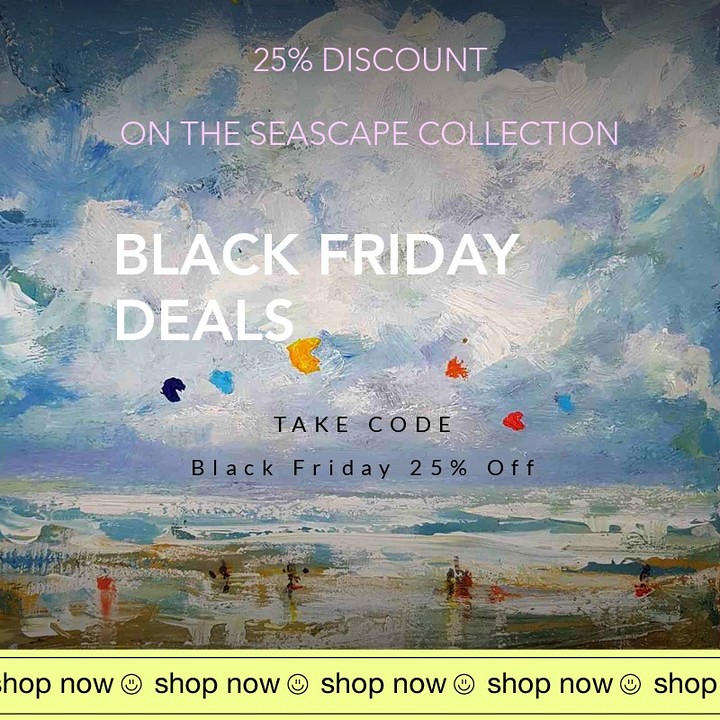This image is a digital advertisement featuring a backdrop that resembles an impressionist-style oil painting. The artwork vividly showcases a seascape where the upper two-thirds of the image is dominated by a sky filled with clouds. The lower third is split between ocean waves lapping onto a sandy shore and various shades of shadows interspersed with streaks of orange and brown. Centered at the top of the image, the text "25% discount" appears in white or light pink, followed by "on the Seascape Collection" slightly below it. Just beneath this, "Black Friday deals" is prominently displayed in larger white text. Lower down, a cursive line somewhat shaped like a heart, adorned with a spectrum of dark blue, yellow, orange, and red hues, adds a decorative touch. Near the bottom, the instruction "Take code BLACK FRIDAY 25% off" is in black text. Finally, a bold yellow banner stretches across the base, repetitively stating "shop now" in black text interspaced with smiley faces, creating a contrasting, albeit eye-catching, call to action.